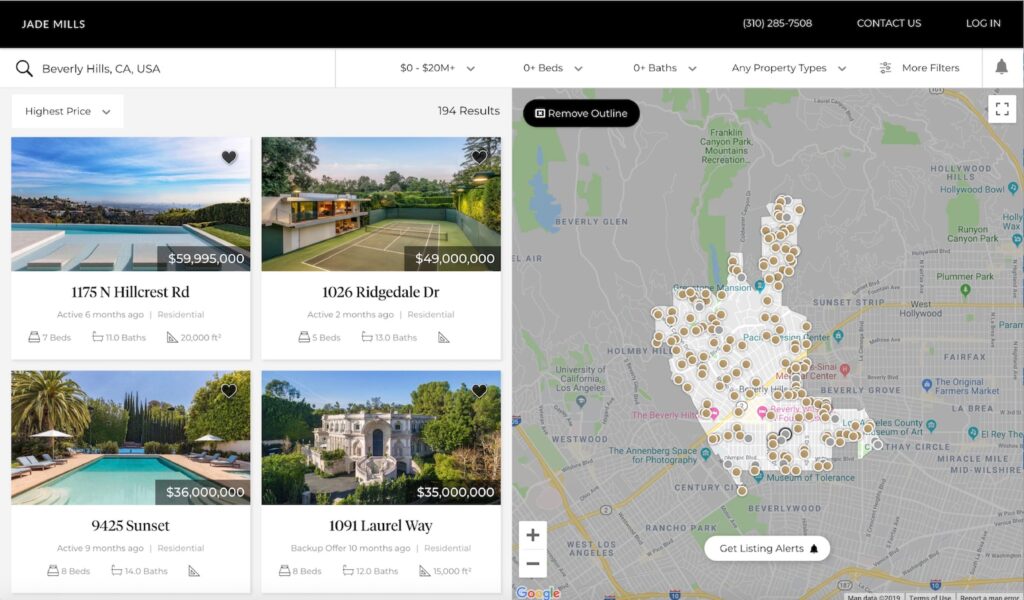The image depicts a real estate website specializing in properties located in Beverly Hills, California, managed by Jade Mills. The website features a prominent black strip stretching across the top, which includes the site name, a contact phone number, a "Contact Us" link, and a login option. The search bar visibly indicates "Beverly Hills, California, USA" as the location, and filters allow users to search for houses within the price range of $0 to $20 million. The drop-down menus let users refine their search by selecting the number of bedrooms, bathrooms, property types, and additional filters.

On the left side of the website, there are listings for four houses, three of which prominently display their outdoor amenities. Two of these houses feature swimming pools, while one boasts a grass tennis court. Each listing includes the property addresses, with one notably located on Laurel Way.

On the right side, the website showcases a map of Beverly Hills. This map provides an outline of the area and highlights the specific locations of houses for sale with small dots. The map itself has a gray background, while the regions with available listings are shown in white.